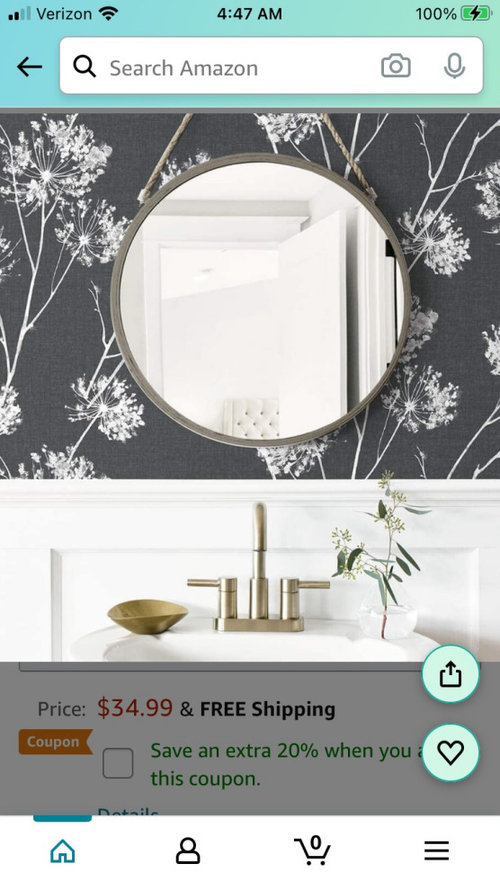A screenshot from an Amazon website is captured at 4:47 AM, as indicated by the timestamp in black at the top right corner. The top portion of the screenshot features a teal-colored status bar. On the left, black service bars and the Verizon label reside next to black Wi-Fi signal strength icons. Completing the top bar content is a 100% battery indicator highlighted by a green full battery icon with a black lightning bolt across it.

Beneath this, a white search bar displays the text "Search Amazon" in black font, flanked on the left by a black left-pointing arrow. 

The image shows a bathroom, centered around a circular mirror against a wall adorned with gray wallpaper featuring white dandelion-like flowers. Below the wallpaper, portions of a white wall are visible, leading to a sink outfitted with brass fixtures.

The price information is prominently displayed, indicating "$34.99" in red, preceded by the word "price" in gray. A black ampersand followed by "free shipping" in black is noted just below. A green text says "save an extra 20%" next to a partially obscured word covered by a green circle featuring a black heart icon. Further, it states "this coupon" in green, with an orange tag labeled "coupon" in white adjacent to it. Above the green circle with the heart, another green circle contains a save icon.

At the bottom of the screenshot, four icons are visible: a green home icon, a black people icon, a black cart icon, and an icon with three horizontal black lines.